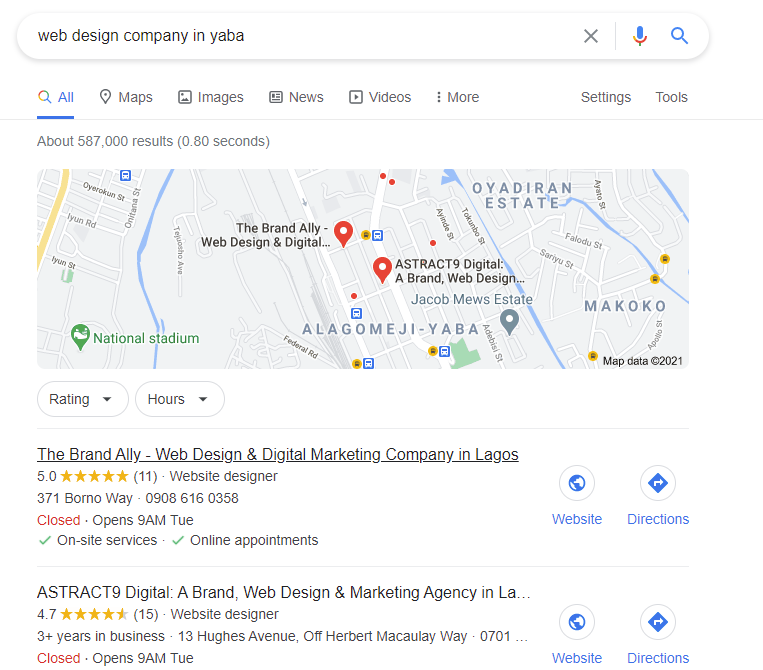The image depicts a website, prominently showcasing a search bar at the top, labeled "Web Design Company in Yabba" (spelled Y-A-B-A). To the right of the search bar, there is an 'X' icon followed by a vertical line, a microphone icon, and a magnifying glass icon. Beneath the search bar, the navigation menu is displayed, starting with "All" in blue, underlined with a blue line, and accompanied by a magnifying glass icon. The menu continues with "Maps," "Images," "News," "Videos," and "More." Further to the right, options for "Settings" and "Tools" are available.

Below the navigation bar, the search results indicate approximately 587,000 results retrieved in 0.80 seconds, displayed in parentheses. The main section reveals a map highlighting various streets, a waterway, and notable landmarks such as the "National Stadium." Two red markers indicate notable locations: "Brand Alley Web Design and Digital" and "Abstract Mind Digital." However, the full name and description of the latter are partially cut off.

On the lower right corner of the map, there is a note stating "Map Data, Copyright 2021." Below the map, there is a section titled "Rating Hours" accompanied by a drop-down menu. Further down, it details information about the "Brand Alley Web Design and Digital Marketing Company in Lagos," followed by details about "Abstract Mind Digital," described as a web design and marketing agency.